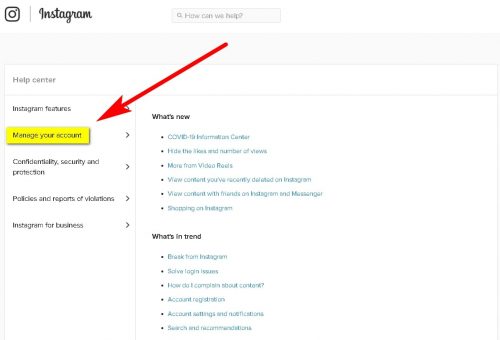The image displays the admin panel for Instagram on a smartphone screen. In the upper left-hand corner, the Instagram logo, rendered in its iconic scripted font, is prominently visible alongside a small camera icon. Below the logo, a vertical menu on the left includes options such as Help Center, Instagram Features, Manage Account, Confidentiality, Security and Protection, Policies, Reports and Violations, and Instagram for Business. The "Manage Account" option is highlighted in yellow and marked with a large red arrow originating from the upper right corner of the screen, directing attention to it.

To the right, there's a section titled "How can we help?" featuring a search bar. Below this, under "What's New," listed in blue font with black bullet points, are the following options: COVID-19 Information Center, Hide the Likes and Number of Views, More from Video Reels, View Content You've Recently Deleted, View Content with Friends on Instagram with Messenger, and Shopping on Instagram.

Additionally, under the "What's in Trend" section, similarly formatted in blue with black bullet points, there are topics such as Take a Break from Instagram, Login Issues, How Do I Complain About Content, Account Registration, Account Settings and Notifications, and Search and Verifications. The text appears slightly blurry and small, but the details are discernable.